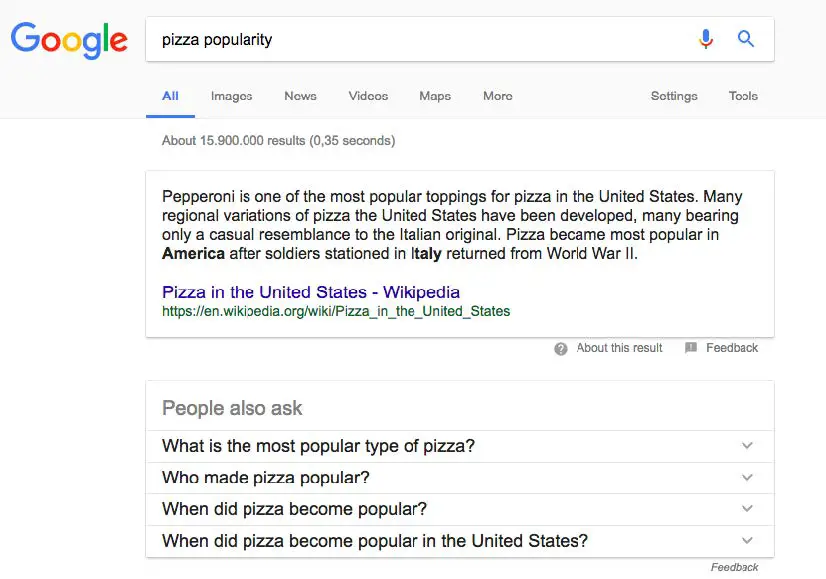In this image, we see a Google search results page displaying information about the popularity of pizza. At the top left, the Google logo is prominently featured in its characteristic colors: blue, red, yellow, blue, green, and red. In the central search field, the query "pizza popularity" is displayed, accompanied by the voice search icon and a magnifying glass icon to the right.

The search categories listed below the search field include: All, Images, News, Videos, Maps, More, Settings, and Tools. The search results indicate there are approximately 15,900,000 results, fetched in 0.35 seconds.

The snippet of text from the search results explains that pepperoni is one of the most popular pizza toppings in the United States. It notes that many regional variations of pizza in the U.S. have evolved, often only loosely resembling the Italian original. It highlights that pizza became extremely popular in America after soldiers stationed in Italy during World War II brought back a fondness for it.

A specific search result from "Pizza in the United States - Wikipedia" provides a link for further information. Additionally, a section titled "People also ask" lists related questions: "What is the most popular type of pizza?", "Who made pizza popular?", "When did pizza become popular?", and "When did pizza become popular in the United States?" 

This detailed description provides a comprehensive view of the Google search results page and the specific details within.